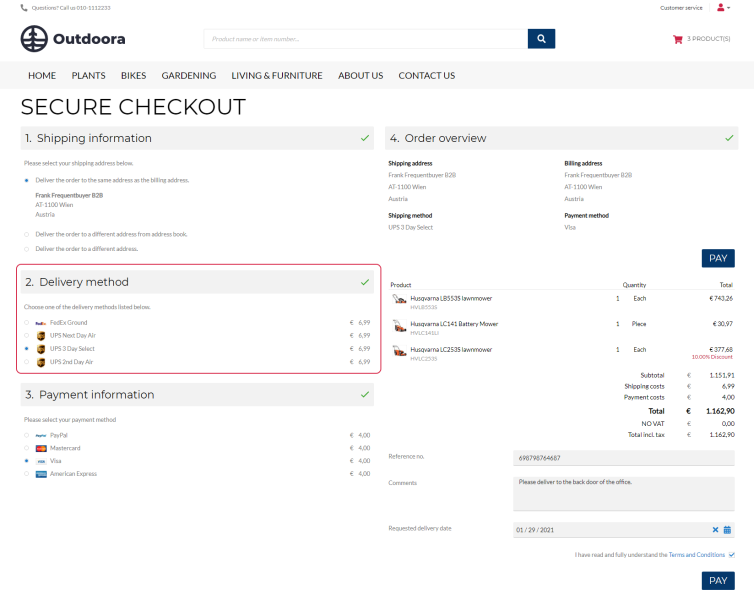Image Caption: 

The top left corner features a phone icon accompanied by text that is too small to read. On the right side, there are additional unreadable text, an icon depicting a person, and a dot next to it. Below, a circle contains a vertical line with arrow-like indicators running from top to bottom, intersected by two horizontal lines, with the text "Out Dora" displayed. 

In the upper section, there's a gray rectangle with smaller text, followed by a blue rectangle with a magnifying glass icon, a red shopping cart, and accompanying text that is too hard to decipher. Another gray rectangle lists categories such as "Home, Plants, Bikes, Gardening, Living, Furniture, About Us, Contact Us." Below this menu, "Secure Checkout" is written in bold uppercase letters.

Subsequently, a gray rectangle labeled "One Shipping Information" appears, adjacent to another gray rectangle labeled "Four Order Overview" with a green check mark at its end. Substantial text underneath remains unreadable. On the left, a red-outlined rectangle encases a gray rectangle labeled "Two Delivery Method," also marked with a green check mark. Below this, more text and images are present but are too small to interpret.

Continuing down, there is a gray rectangle labeled "Three Payment and Information" with a green check mark. Beneath this are words and symbols representing various payment methods, accompanied by a blue dot and more illegible numbers.

Towards the right, a prominent blue rectangle seems to say "Pay," and additional text and symbols on both sides are again too small to discern, including some red text underneath. More words and numbers follow.

In the bottom section, there are alternating gray rectangles and words, with some gray rectangles appearing to contain dates. A blue ‘X’ and a blue calendar icon are on the right-hand side, with nearby text in black and blue, accompanied by a check mark and another blue rectangle reading "Pay."